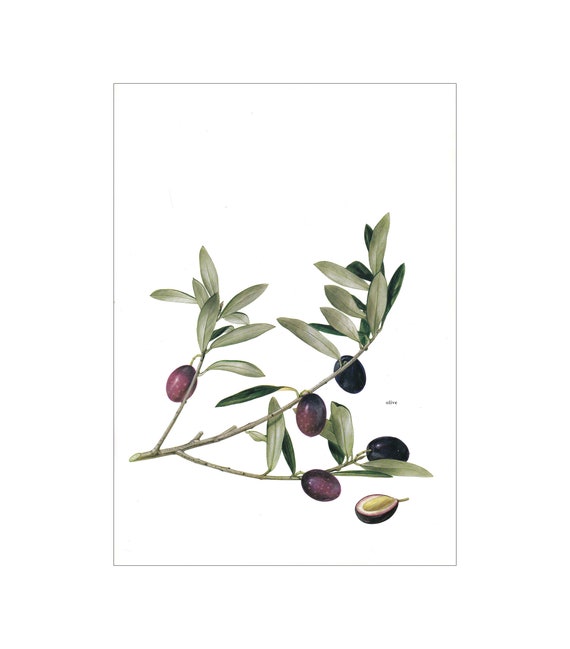The image appears to be a detailed illustration or painting set against a white background, resembling a note card. The upper third of the note card is empty, and the image begins about a third of the way down. The illustration features an olive twig with three distinct branches, each adorned with medium to dark green leaves of varying shades. 

The left branch bears a single olive, while the middle branch displays two olives, and the bottom right branch also holds two olives. Below these branches, at the very bottom right of the image, there's a split olive turned upward, revealing its inner flesh. The olives exhibit a color spectrum ranging from light purple to a deep, almost black hue. The entire image is framed by a grey, border-like outline. Additionally, on the lower right-hand side, there is a small, black text signature, which likely says "olive."